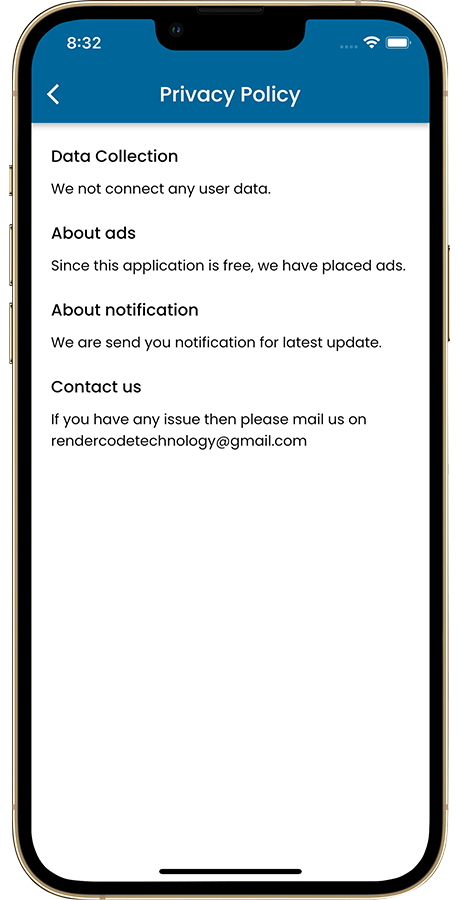In this image, we see a screenshot from an iPhone displaying a "Privacy Policy" page. The top of the page features a blue border with white text that reads "Privacy Policy." In the top-left corner, there is a back arrow, indicating this is a submenu page.

The page is divided into several sections with headlines and brief descriptions, though the English text contains several grammatical errors. The first section, titled "Data Collection," states "We not connect any user data." The intended message likely was "We do not collect any user data."

The next section is "About Ads," which mentions that the application is free, so ads have been placed within it.

Following that, the section "About Notification" reads, "We are send you notification for latest update," which should be corrected to "We will send you notifications for the latest updates."

Finally, the "Contact Us" section provides an email address for inquiries: "RenderCodeTechnology@gmail.com," with the note, "If you have any issue, then please mail us."

Overall, while the information is fairly clear, it is evident that the text was authored by someone with limited proficiency in English.